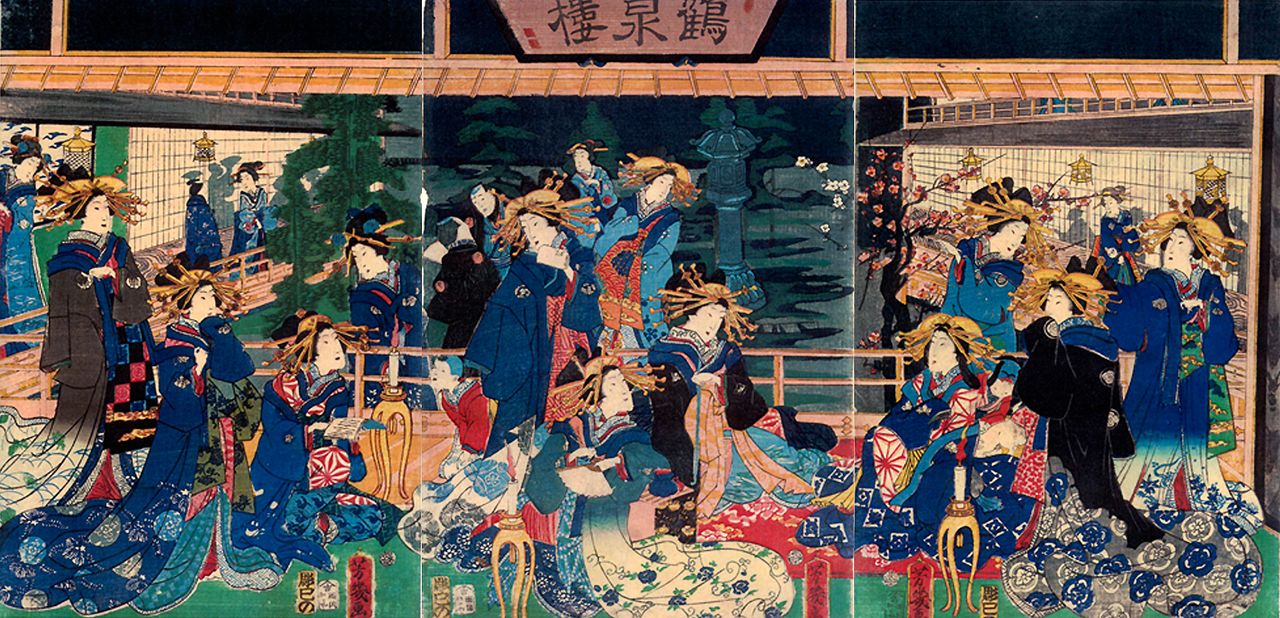This piece of traditional Japanese art is a detailed triptych that, when assembled, forms a cohesive and elaborate scene. The top section of the artwork features a banner or sign with Japanese characters, set against a plum-colored background. Below this banner, the scene unfolds inside a beautifully depicted building, accented with orange and black panels at the roof.

The central image is populated by numerous figures, likely geisha, adorned in exquisite silk robes that predominantly feature bright blues, reds, and various intricate patterns. Their elaborate gold headdresses and white-painted faces add to the grandeur of the scene. Some of these women stand while others sit, set against a lush backdrop that includes trees, statues, greenery, and flowers—contributing to the garden-like atmosphere.

The artwork is segmented into three distinct panels, with visible seams indicating their separation, yet they come together seamlessly to present a lively and vibrant tableau. Screens flanking the sides and a courtyard hinted in the center evoke the elegance of traditional Japanese architecture, immersing the viewer in a beautifully rendered, culturally rich moment.